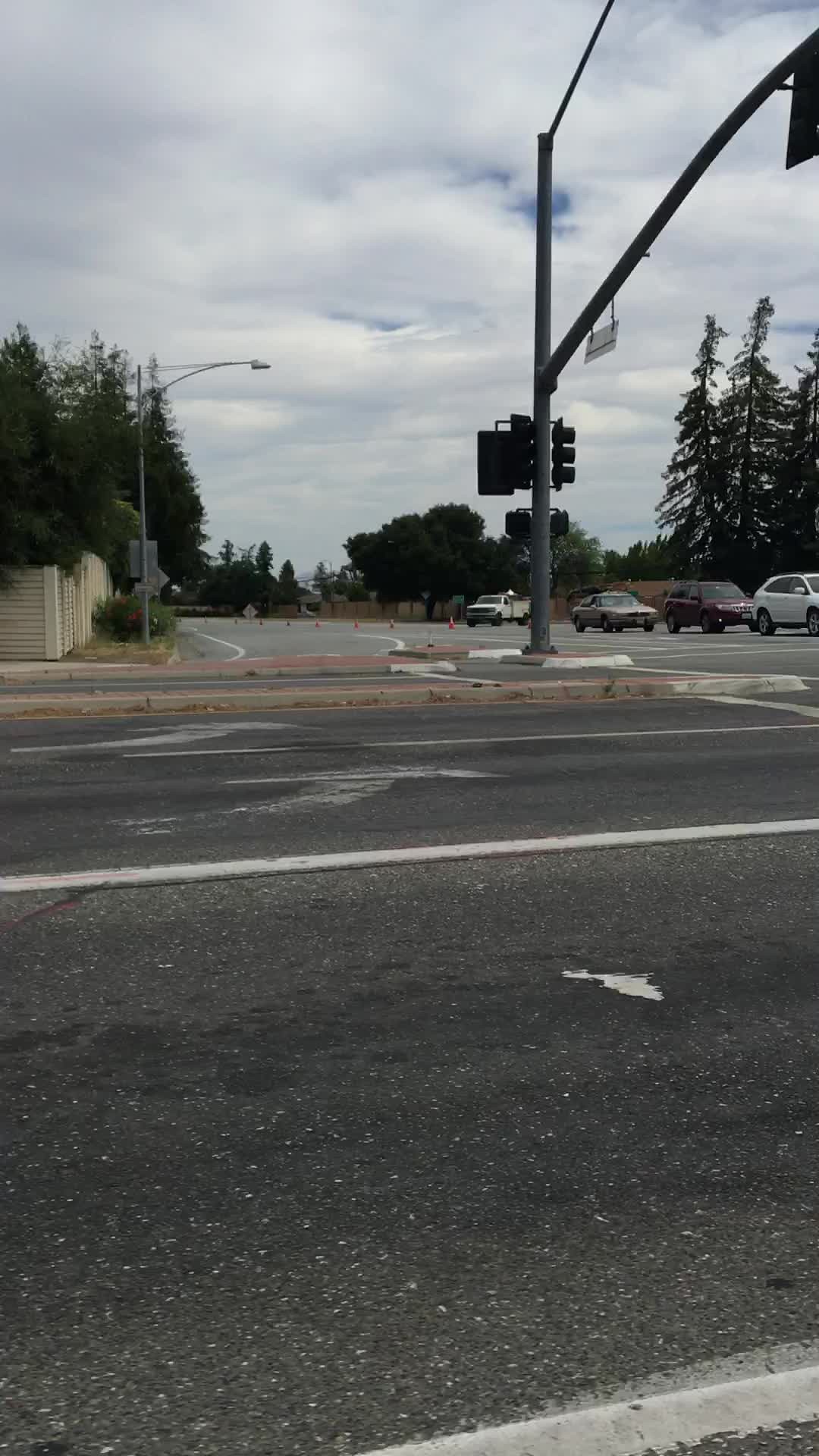This image captures a bustling urban street scene. The black asphalt of the road is prominently marked with white lines indicating lanes, and there is a noticeable spillage staining the middle of the street. Two large white arrows designate a left-turn lane. A streetlight mounted on a pole stands on the near side, accompanied by an indistinct street sign. Across the street, another light pole stands beside a fence adorned with some trees, further enhancing the scene. Above, the sky is mostly overcast with thick clouds allowing only a glimpse of blue. The far side of the street is lined with more trees and also features a wooden fence. Scattered along the street are some orange cones, possibly indicating construction or maintenance work. Vehicles are present, including a white car, a red car, and a goldish-tan car, with a white truck further in the background near the wooden fence. The overall atmosphere is one of a typical city street teeming with subtle details.